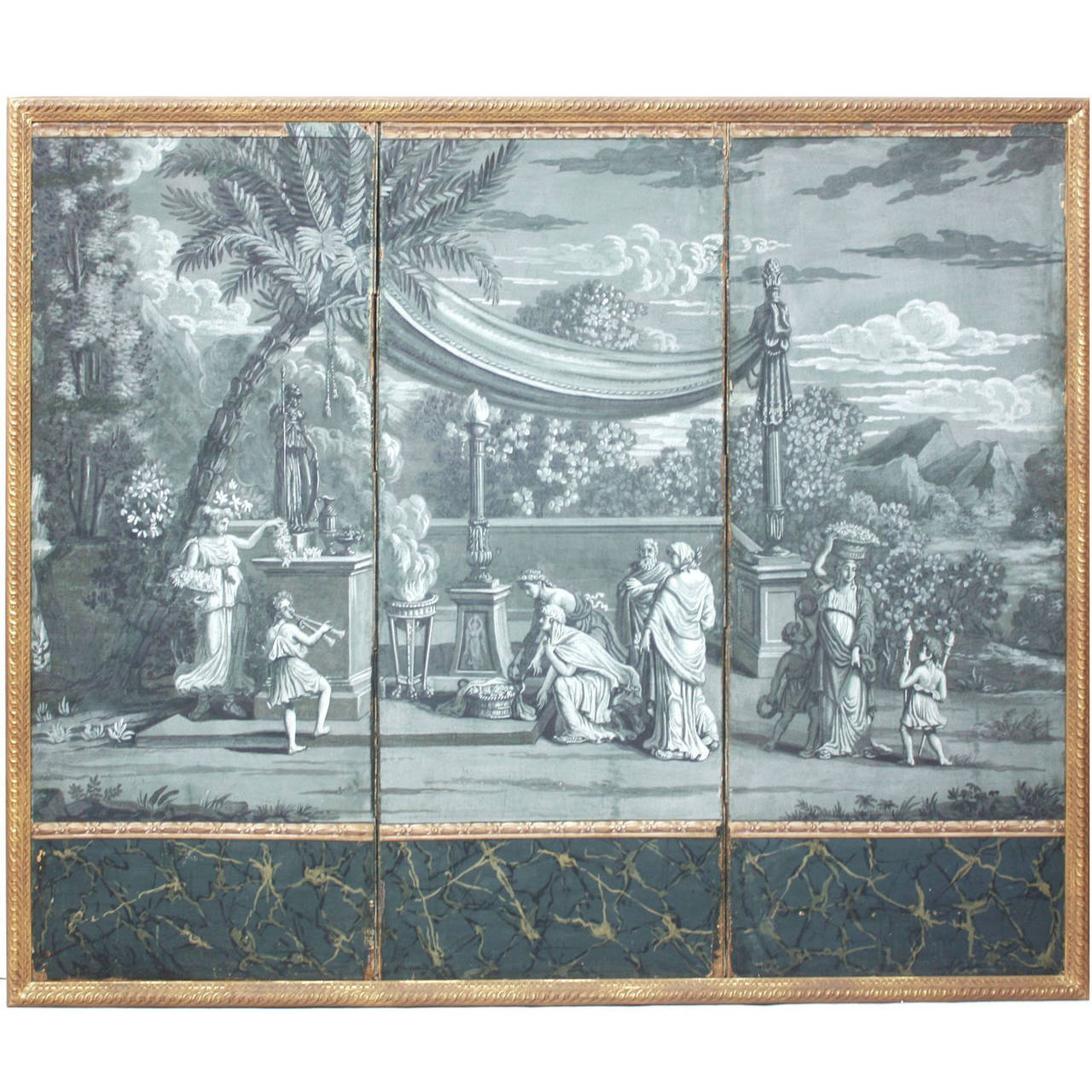This captivating piece of art, framed elegantly in gold, presents a grayscale depiction of a serene Grecian garden, reminiscent of ancient Greek or Roman times. The setting radiates an aura of paradise with tall palm trees leaning as if swayed by a gentle breeze under a sky adorned with wisps of dark gray clouds. Among the figures in this tranquil outdoor courtyard, some are dressed in flowing robes, evocative of classical attire, while children play. A notable feature is a young girl dancing, another playing a flute, and a woman balancing a basket on her head. The scene is set against a textured, marble-like base in shades of black, white, gray, and a hint of brown, giving the artwork a timeless, washed-out appearance. This portrayal, void of any text, offers a glimpse into an idyllic, bygone era, caught in the essence of leisure and beauty.